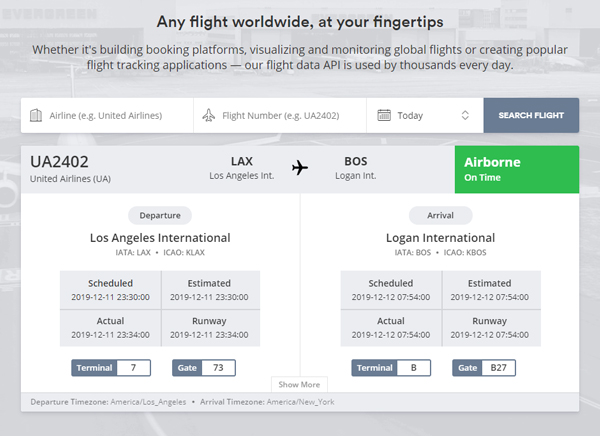The image showcases a detailed pop-up window titled "Any Flight Worldwide at Your Fingertips," prominently placed at the top center in black font. Below the title, a smaller text elaborates on the various applications of their flight data API, stating: "Whether it’s building booking platforms, visualizing and monitoring global flights, or creating popular flight-tracking applications, our flight data API is used by thousands every day."

Beneath this text, a segmented bar divided into four sections includes areas for inputs: "Airline" on the far left, followed by "Flight Number," "Today," and a "Search Flight" button on the far right. 

Directly below this bar, a detailed chart for flight information is displayed with the heading "UA2402, United Airlines" on the top left. Centrally, it indicates the route "LAX to BOS" (Los Angeles International Airport to Boston Logan International Airport). To the right, a green-highlighted segment announces that the flight is "Airborne On Time."

The chart is further divided into two sections: "Departure" on the left and "Arrival" on the right. The departure section includes comprehensive details for Los Angeles International Airport, featuring fields such as Scheduled, Estimated, Actual, and Runway times, along with Terminal 7 and Gate 73. The arrival section mirrors this format for Logan Airport, including Scheduled, Estimated, Actual, and Runway times, designating Terminal 8 and Gate B27.

In the footer, affiliations with the NASA Jet Propulsion Laboratory and the California Institute of Technology are noted.